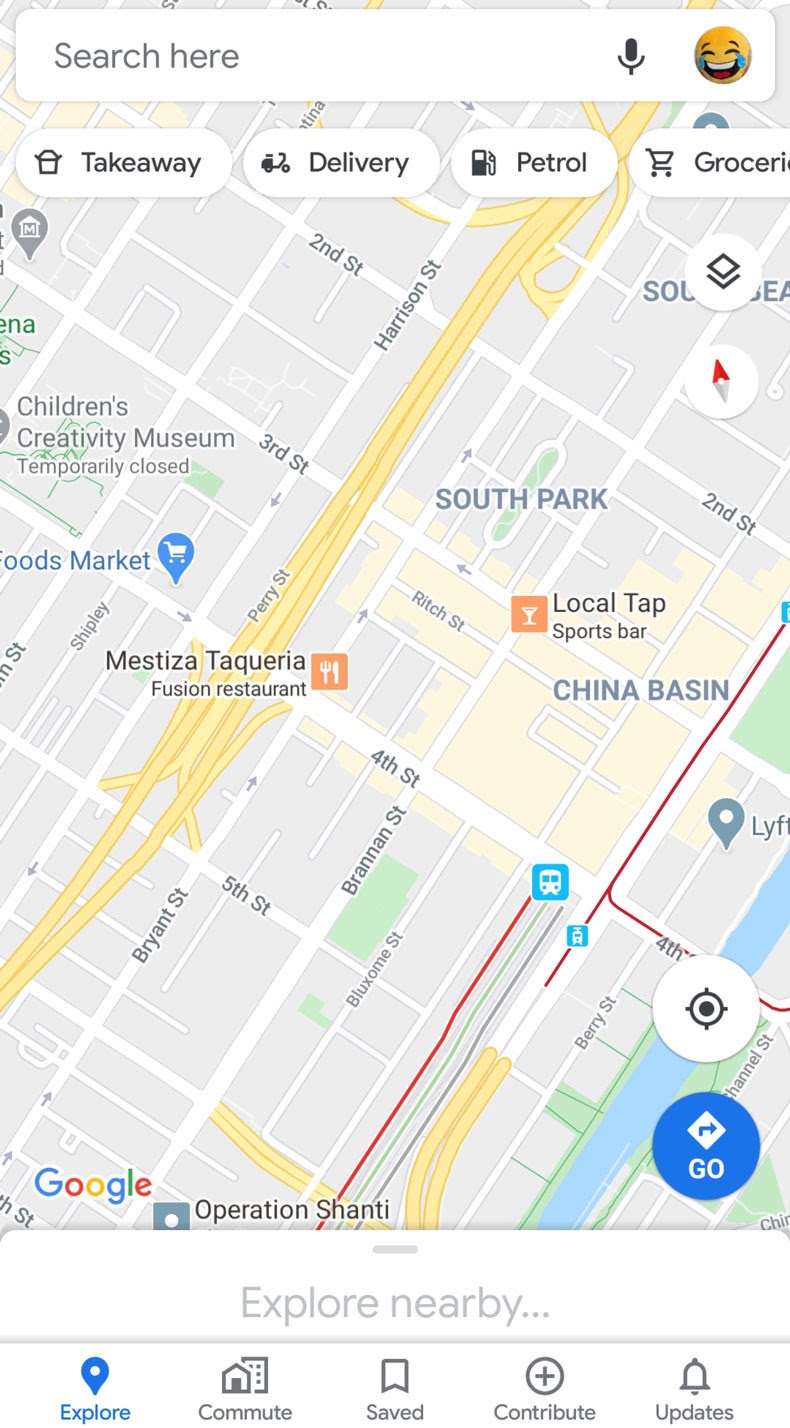This image appears to be a Google Maps screenshot taken on a smartphone. The topmost section features a search bar labeled "Search here," accompanied by a microphone icon and an emoji of a laughing face with tears. Just below the search bar, there is a quick access menu with options for "Takeaway," "Delivery," "Petrol," and "Grocery."

The map itself is centered around a city area, likely indicated by numbered streets including 2nd Street, 3rd Street, 4th Street, and 5th Street, all intersected by an expressway. Specific neighborhood names, such as China Basin and South Park, are visible. Notable locations include the temporarily closed Children's Creativity Museum.

Various points of interest and establishments are prominently marked on the map. These include Mestiza Tangaria, the Fusion Restaurant, Local Tap Sports Bar, Operation Shanty, and what appears to be a Lyft pickup or station location. The map also features a directional compass icon showing the orientation (north-south).

At the bottom of the screen, there are several navigation buttons labeled "Explore," "Commute," "Saved," "Contribute," and "Updates," allowing the user to switch between different functionalities of Google Maps.